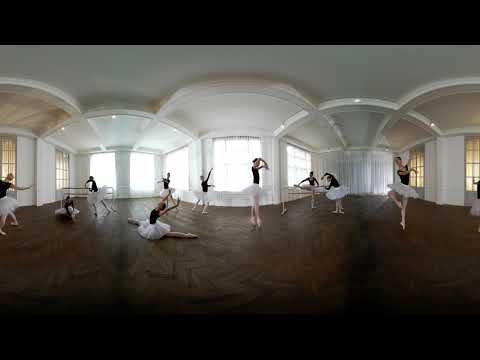The panoramic image captures a bustling ballet studio adorned with intricate architectural details. The dark brown, shiny wooden floor contrasts beautifully with the white-curved, artfully designed ceiling, which features crown molding and elaborate artistic elements. The studio's white walls are punctuated by large windows framed in wood, draped with white curtains. Natural sunlight pours in through these windows, casting a warm glow across the room, while softer, brownish lights filter through the side windows.

In the center of this dynamic scene, numerous ballerinas in action populate the space, all dressed in elegant white tutus and black tops. Each ballerina strikes a unique pose amidst their collective dance—some pirouetting, some with legs raised, arms uplifted, and a couple engaged in floor splits. The image captures the fluidity and diversity of their movements, perfectly showcasing the lively energy and grace of a ballet performance in an exquisite setting.